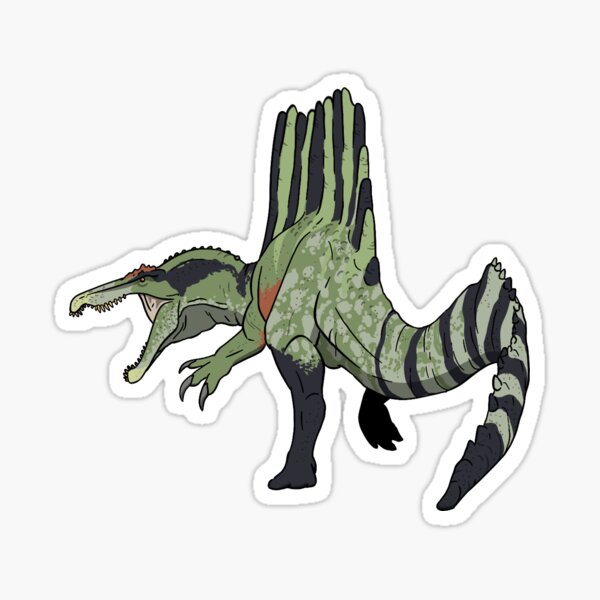The image showcases a detailed depiction of a spinosaurus dinosaur sticker. The spinosaurus, a notably large dinosaur, is portrayed standing on its hind legs with its front legs raised, each bearing three phalanges tipped with long green claws. The dinosaur's body is primarily colored in shades of green and brown, featuring a camouflage-like pattern with stripes alternating between dark green, light green, and white along its back and tail. Distinctively, it has a long narrow snout, an open mouth displaying sharp teeth, and a prominent sail-like structure on its back. The sticker is outlined with a white border and contains no additional text. The creature is oriented with its head facing left and its elongated tail pointing towards the bottom right, with an array of colors including touches of dark orange, light tan, and hints of light yellow on the snout, enhancing its detailed and vivid appearance.